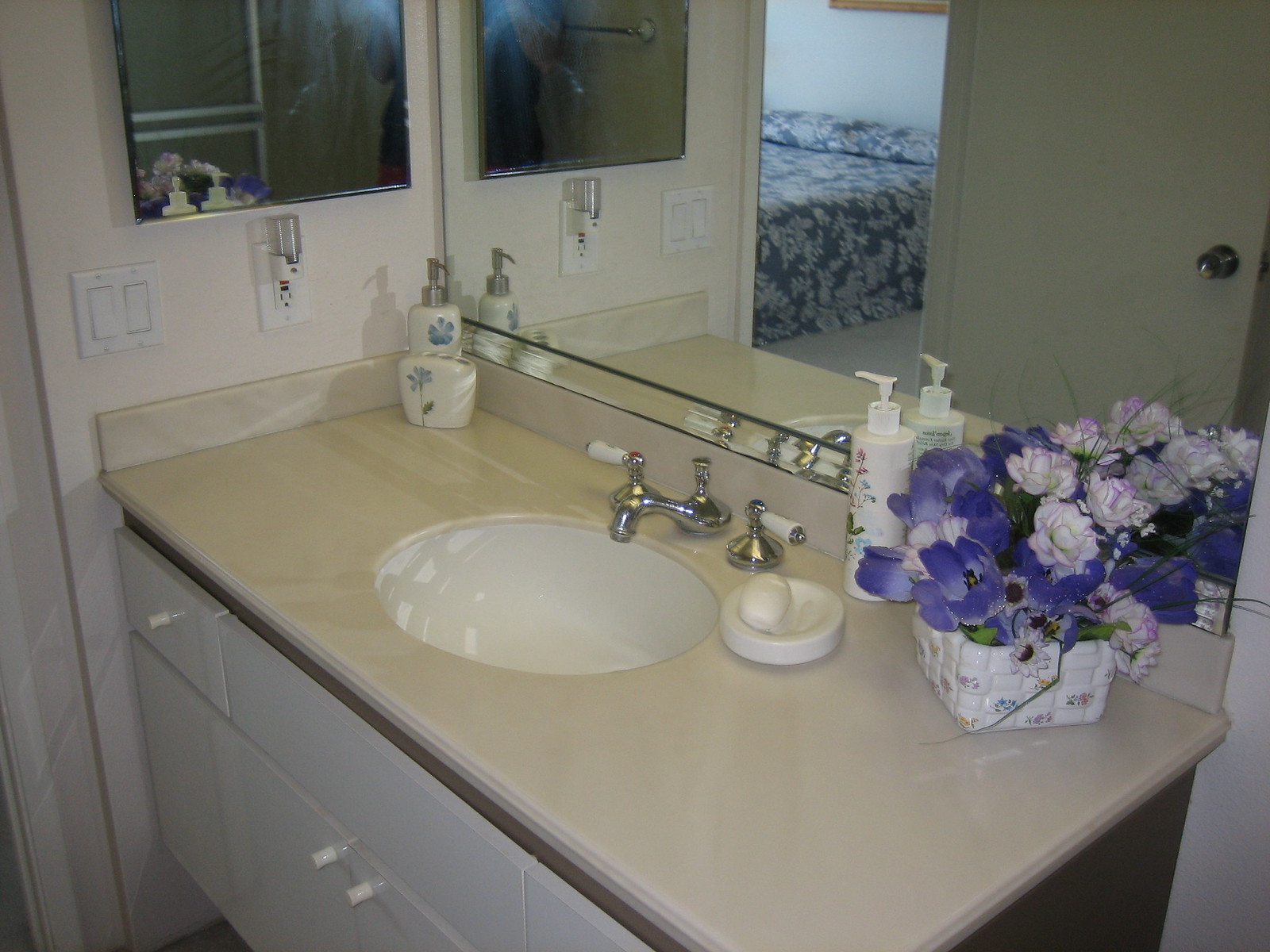This photograph shows a neatly arranged bathroom sink within what appears to be a sizeable vanity setup, possibly in a home or a hotel. The centerpiece is a sleek, white inset sink set into a wide, light tan vanity. The vanity, which seems to be painted wood, features two central drawers beneath the sink and additional pull drawers on each end for ample storage. 

To the right of the sink, a charming flower bouquet beside a white wicker basket adds a touch of elegance and homeliness. Also positioned on the right is a bottle of lotion or soap. On the left side, another squirt bottle and an empty toothbrush holder are neatly placed. 

A nightlight plugged into the GFCI outlet to the left of the sink provides a functional touch. Above the vanity, there are mirrors in both the front and side positions, offering comprehensive reflection options. Two switches, presumably for lighting and other utility controls, are mounted to the left of the mirror. The entire setup, from the chrome-finished hot water faucet to the meticulous arrangement of elements, suggests a well-thought-out design aimed at both utility and aesthetic appeal.